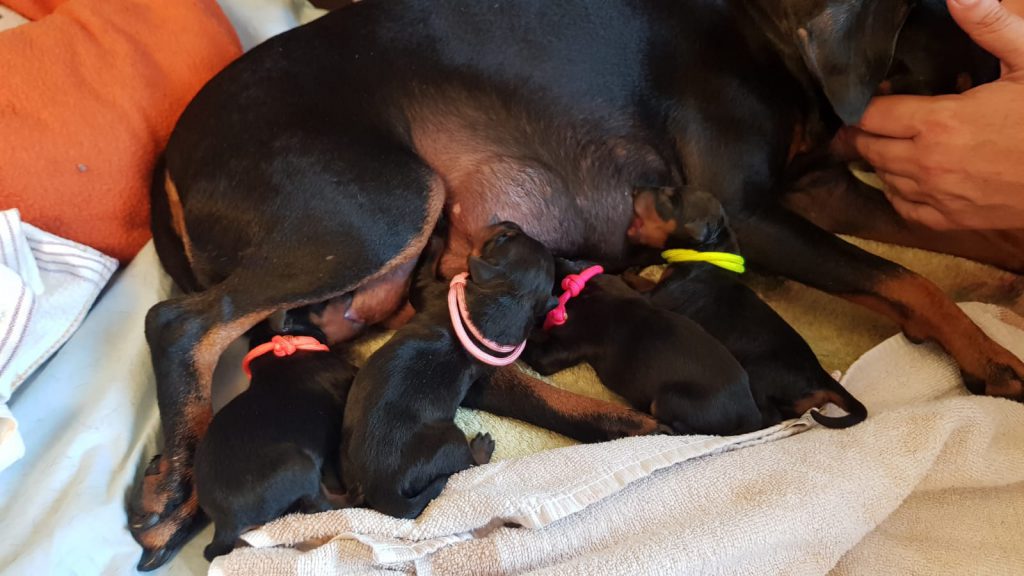The photograph captures a tender moment of a mother dog, likely a Rottweiler, surrounded by four nursing puppies. The scene is set on a white towel and a soft yellowish mat, emphasizing the clean and cozy environment. The mother dog, distinguishable by her black fur and brown paws, is being gently petted by a human hand, which is visible only partially. The puppies, all black with brown paws, are adorned with different colored makeshift collars—orange, pale pink, hot pink, and lime green—for identification. They nurse diligently, each seeking nourishment. Surrounding the family are various blankets, pillows, and towels, including a prominent rolled-up orange blanket behind the mother, adding a splash of color to the serene setting.